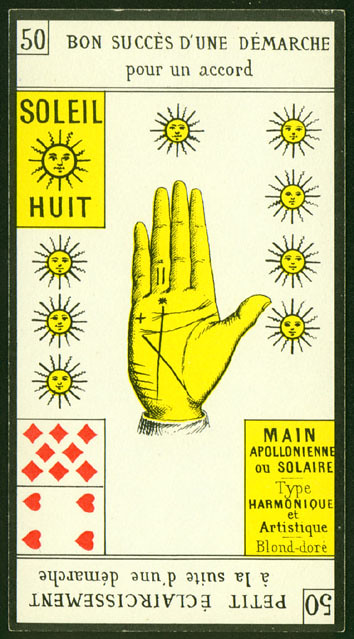Poster Description:

The poster, predominantly in French, features a visually striking centerpiece - a yellow hand with fingers closed together. This hand is marked with lines and arrows reminiscent of a palm reading, showcasing the number "11" on the ring finger and a plus sign on the right side of the palm.

At the top left corner, the number "50" indicates a cost of 50 cents. The text "Bon Success Dune de Marche Pour Un Accord Soleil Huit" suggests a theme of good success with some form of agreement under the sun. Surrounding this inscription are nine smiling sunshines, each adorned with facial features, radiating from the center with squiggly sun rays.

Beneath this, on the left side, is a playing card motif featuring an "Eight of Diamonds" above a "Four of Hearts". On the right side of the hand, a French phrase reads "Main Apollonienne au Solaire Type Harmonique et Artistique Blondeur", which hints at a blend of harmonic and artistic qualities, potentially related to Apollo, the Greek god of the sun and the arts.

At the very bottom of the poster, upside-down text reads "Petite Eclairissement à la suite d'une démarche", roughly translating to "Small enlightenment following a procedure".

The background of the poster is a creamy color, providing a subtle yet harmonious setting for the vivid illustrations and text.